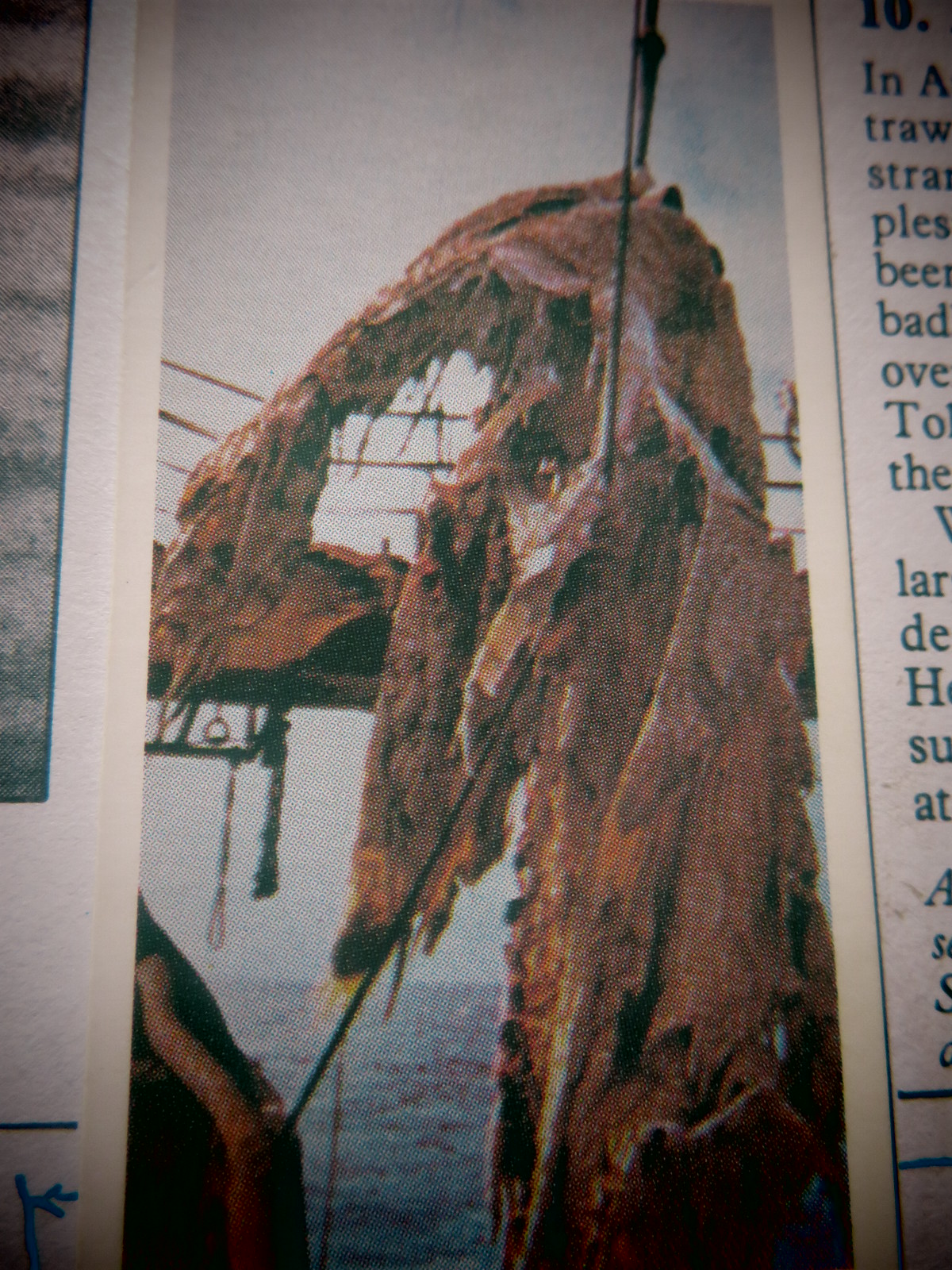The image appears to be a close-up photograph of a magazine or newspaper clipping. The text on the right side is largely illegible, displaying only fragments of words in black and white. The left side features another partially cut-off image. The main image at the center foreground depicts a large object being hoisted from a body of water, likely an ocean or lake, given the visible expanse of water. This object, which appears damaged and tattered, is suspended by cables attached to a red metal structure resembling a bridge with a guardrail. The object itself is fibrous and inconsistent in shape, predominantly orange, resembling a heavily rusted structure or material, possibly debris from a shipwreck or a destroyed raft. The scene lacks a visible horizon and any accompanying text or headlines providing further context.